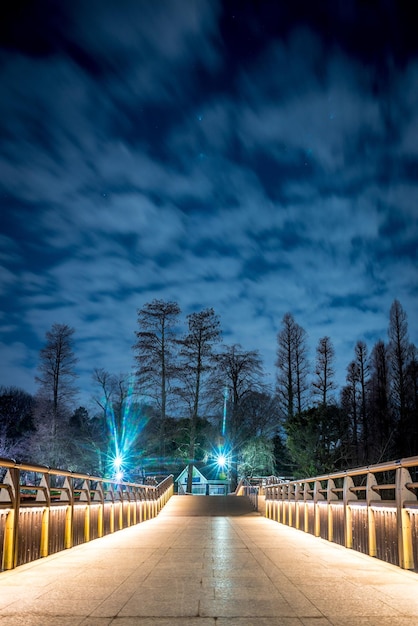The photo captures a nighttime scene of a long, illuminated walkway or bridge with a tiled floor and railings on both sides. The bridge, which appears brown and gold, stretches out towards a distant white house with a dark roof, accentuated by two bright lights. Tall trees, some with sparse foliage and dark green hues, frame the background, hinting at either late fall or winter. The sky above is a deep, dark blue, adorned with a few scattered stars and streaks of clouds, suggesting it might be a long exposure shot, adding an artistic effect with a slightly brighter, almost ethereal appearance of the sky. The overall scene exudes a serene yet mysterious atmosphere, amplified by the glowing lights along the bridge.